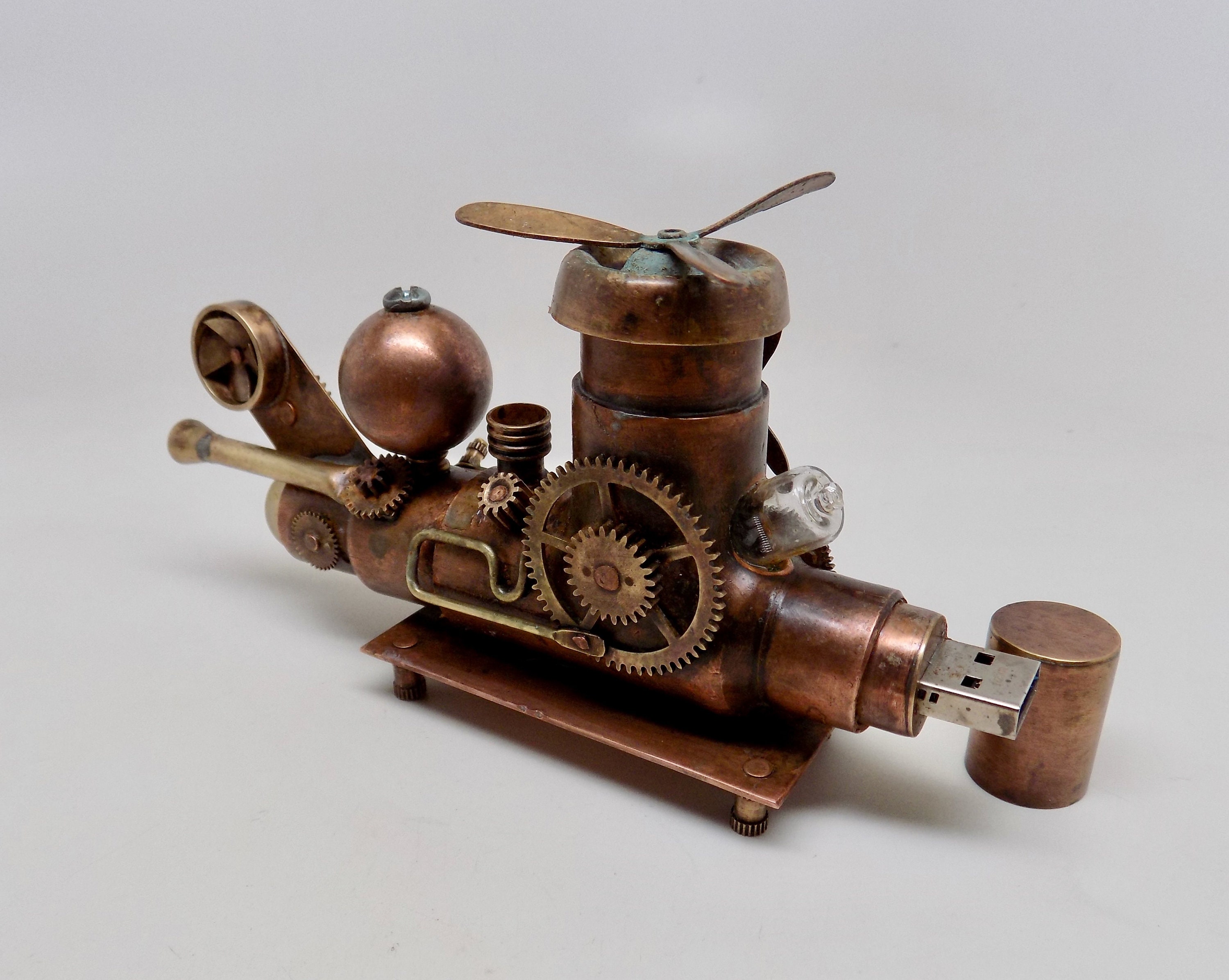In the center of the image, there is a single, unique object against a light gray background. The object appears to be a USB flash drive, designed to look like a mechanical device from the 1800s. It features a metallic, bronze-colored body with a shiny, dark brown finish, resembling old machinery. 

At one end, there is an obvious USB female port, partially covered by a cylindrical cap that appears to provide protection. The device has several intricate details including various-sized gears on its side, a central raised section with three fan-like rotating blades or wings, and a bow-shaped screw. There's also a crank mechanism at the back, similar to what you might find on a tire jack, suggesting an interactive component although it likely isn’t motorized.

The base is a rectangular, golden platform with an orange-copper hue, giving the entire setup a vintage aesthetic. Another notable feature is a seemingly transparent cap over a cylindrical item, possibly another part of the USB port protection. The colors of the object combine elements of brown, gray, white, and black, adding to its antique appearance. The background remains plain with no text or living elements, keeping the focus entirely on the intriguing, steampunk-styled flash drive.